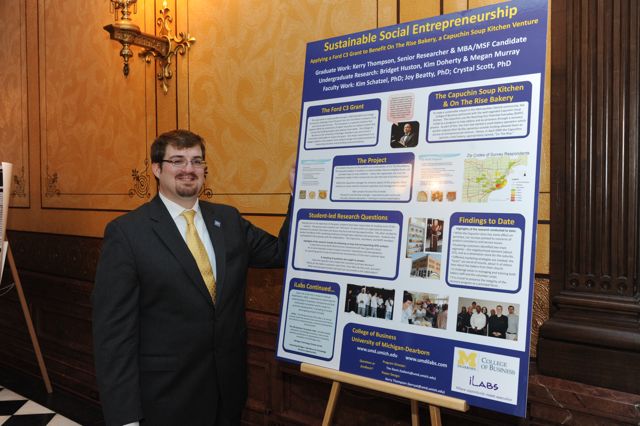In this indoor image, likely taken in a sophisticated venue such as a fancy hotel or possibly a Capitol building, a man is positioned on the left side of the frame. He sports a refined appearance, wearing a black suit, a white dress shirt, and a golden yellow tie accented by a pin on his left collar. His facial features include glasses, brown hair, a mustache, and a brown goatee. He is engaging with a large blue and white sign mounted on a wooden tripod stand on his right, his left hand resting on or pointing towards it for emphasis.

The sign prominently reads "Sustainable Social Entrepreneurship" at the top, and below, in smaller fonts, details various segments. The central section of the sign is divided into six rectangular areas, each containing titles, paragraphs of text, and pictures of people. Specific mentions include information about institutions like the Capuchin Soup Kitchen and On the Rise Bakery. The overall setting is further characterized by elegant elements such as brass lights, additional easels, and a distinct diamond-patterned black and white tiled floor. A substantial black post, likely a support structure, extends towards the ceiling, adding to the grandeur of the environment.